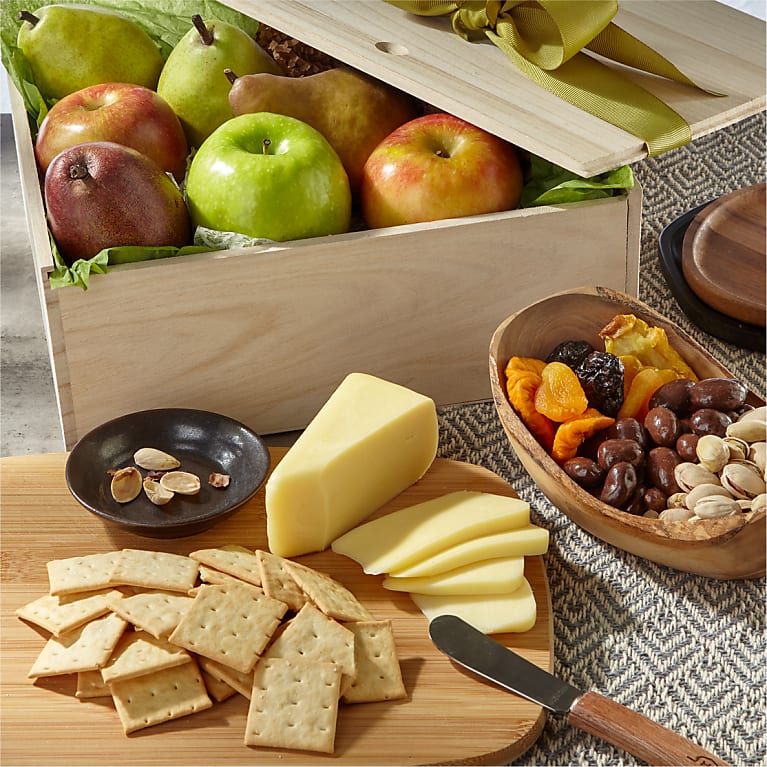In this detailed image, a rustic kitchen scene is meticulously captured. Dominating the upper part of the photograph is a natural wooden crate box, crafted with a lid that is ajar and adorned with a yellow ribbon and bow. Inside the box, nestled in green tissue paper, is an array of fruits: two green pears, two red apples, a green apple, a brownish pear, and a reddish fruit that could be either a papaya or another type of red pear. The crate is positioned on a gray and navy placemat featuring a pattern of squares.

In front of the box, on the right-hand side, there is a small wooden bowl filled with a mix of cashews, prunes, dates, olives, and pistachios. To the lower left of the frame, we see a wooden cutting board acting as a charcuterie board. On this board, there is an assortment of square white crackers, a block of cheese from which four slices have been cut, and a cheese knife resting on the board. Additionally, a black plate nearby holds a few peanut shells. The careful arrangement suggests a setting prepared for an inviting and freshly curated snack or gift presentation.